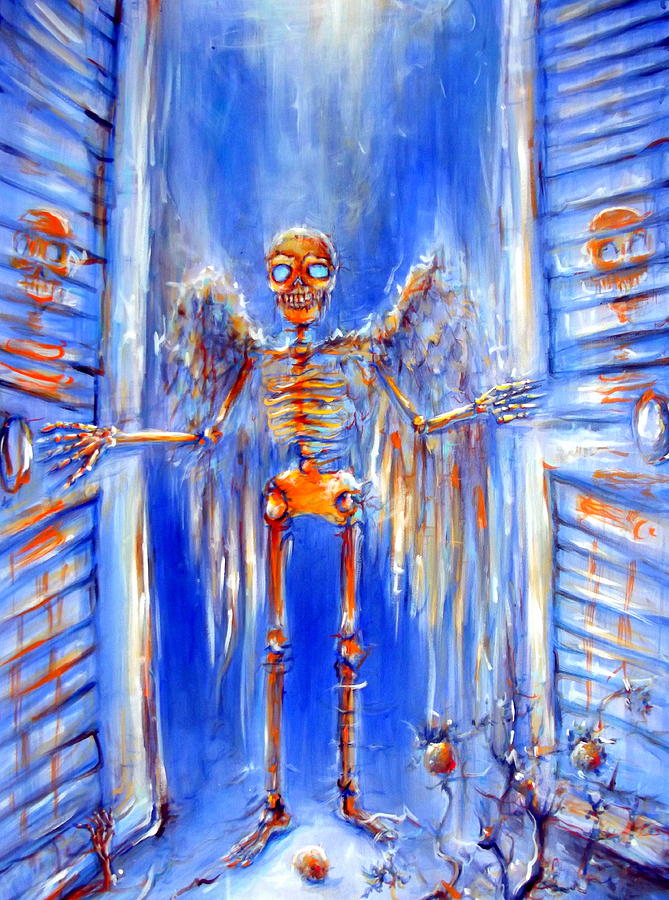The artwork is a detailed painting of a hauntingly beautiful skeleton standing in the center of a doorway. Its eye sockets glow with bright blue light, devoid of pupils, making a striking contrast against the primarily orange and reddish-brown hues of the bone structure. The skeleton is adorned with angelic white wings, touched subtly with shades of blue, orange, red, and gray. It stands amidst a vinyl siding-like wall, accentuating the doorway's structure. Horizontal slatted doors with little knobs, tinted in white and blue undertones, flank the skeleton on both sides, each door bearing an orange depiction of a skeleton, mirroring the central figure. A mysterious white light emanates from above, casting an ethereal glow downwards. At the bottom right corner, a jagged, dark gray plant with round orange fruits grows, adding an intriguing organic detail to the composition. The background is predominantly blue, enhancing the spectral and surreal ambiance of the scene.